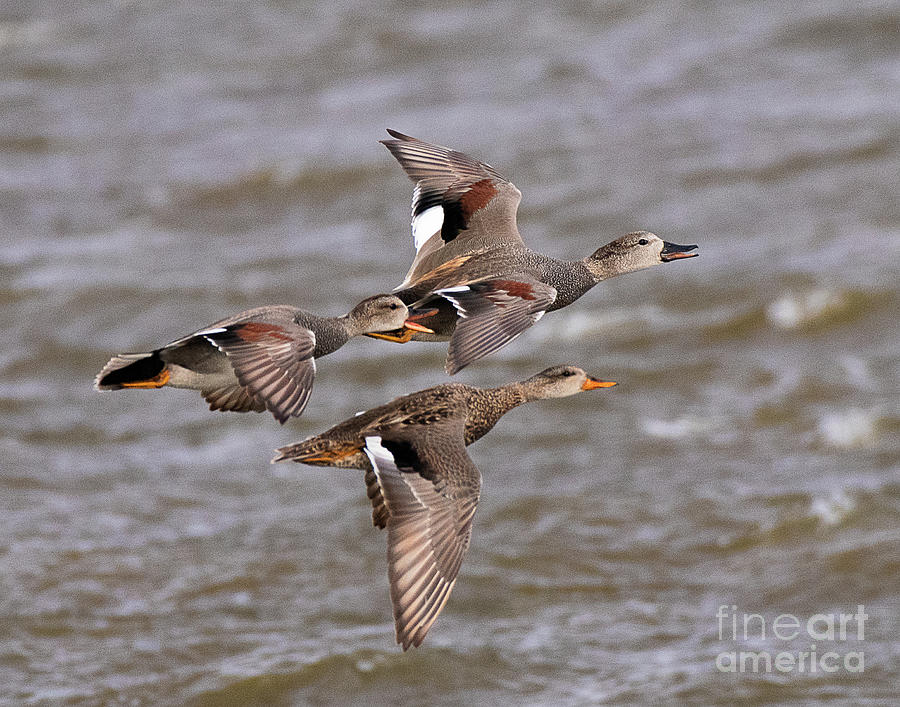This detailed photograph, watermarked by Fine Art America in the bottom corner, captures a vivid scene of three ducks mid-flight over a murky, grayish-brown body of water, marked by subtle waves. The ducks, showcasing a striking variety of colors including shades of brown, tan, black, and white, feature distinctive orange feet and mostly orange beaks, except for one with a black beak. The close-up shot reveals intricate feather details, despite the image's slightly grainy texture. Two of the ducks appear to have their beaks partially open, adding a dynamic sense of motion to the scene, while their expressive eyes are clearly visible, adding to the overall impact of this striking and meticulously captured moment.